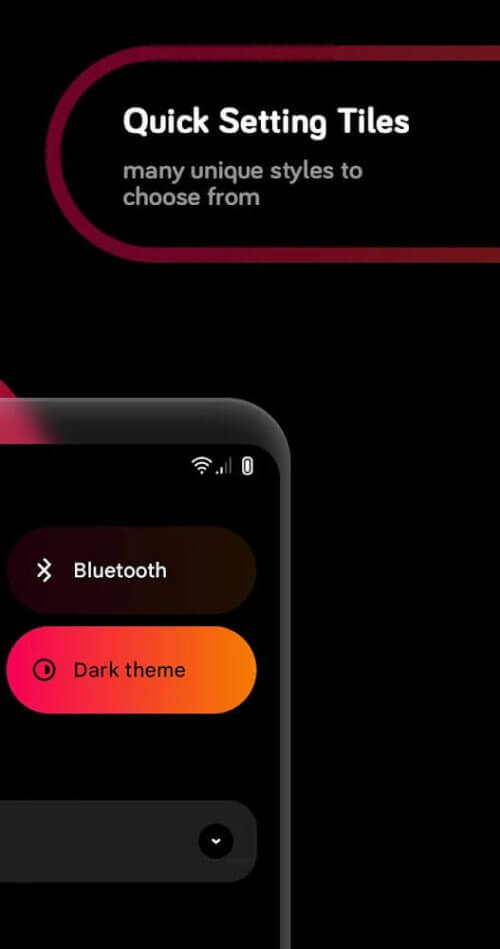The image, designed for mobile viewing, features a predominantly black background, contributing to its sleek and modern aesthetic. In the bottom left corner, there's a graphic of a smartphone with a slightly opaque gray edge. A prominent diagonal pink bar runs from left to right behind the phone, adding a dynamic touch.

The phone's screen is dark, displaying a Wi-Fi icon with two out of four bars and a battery icon indicating it is charging. Two prominent buttons dominate the screen. The first button, a dark orange-gray hue, is labeled "Bluetooth" in white text. Below it, another button labeled "Dark Theme" features a stunning gradient that transitions from pink on the left to a yellowish-orange on the right.

Beneath these buttons, there is a grayish bar with a circular icon and a white arrow pointing downward. At the top of the display, an oval shape with a thick dark red border houses bold white text that reads "Quick Setting Tiles," accompanied by smaller gray text underneath stating, "Many unique styles to choose from." This meticulous arrangement of elements provides a detailed, visually appealing mockup of a smartphone interface.